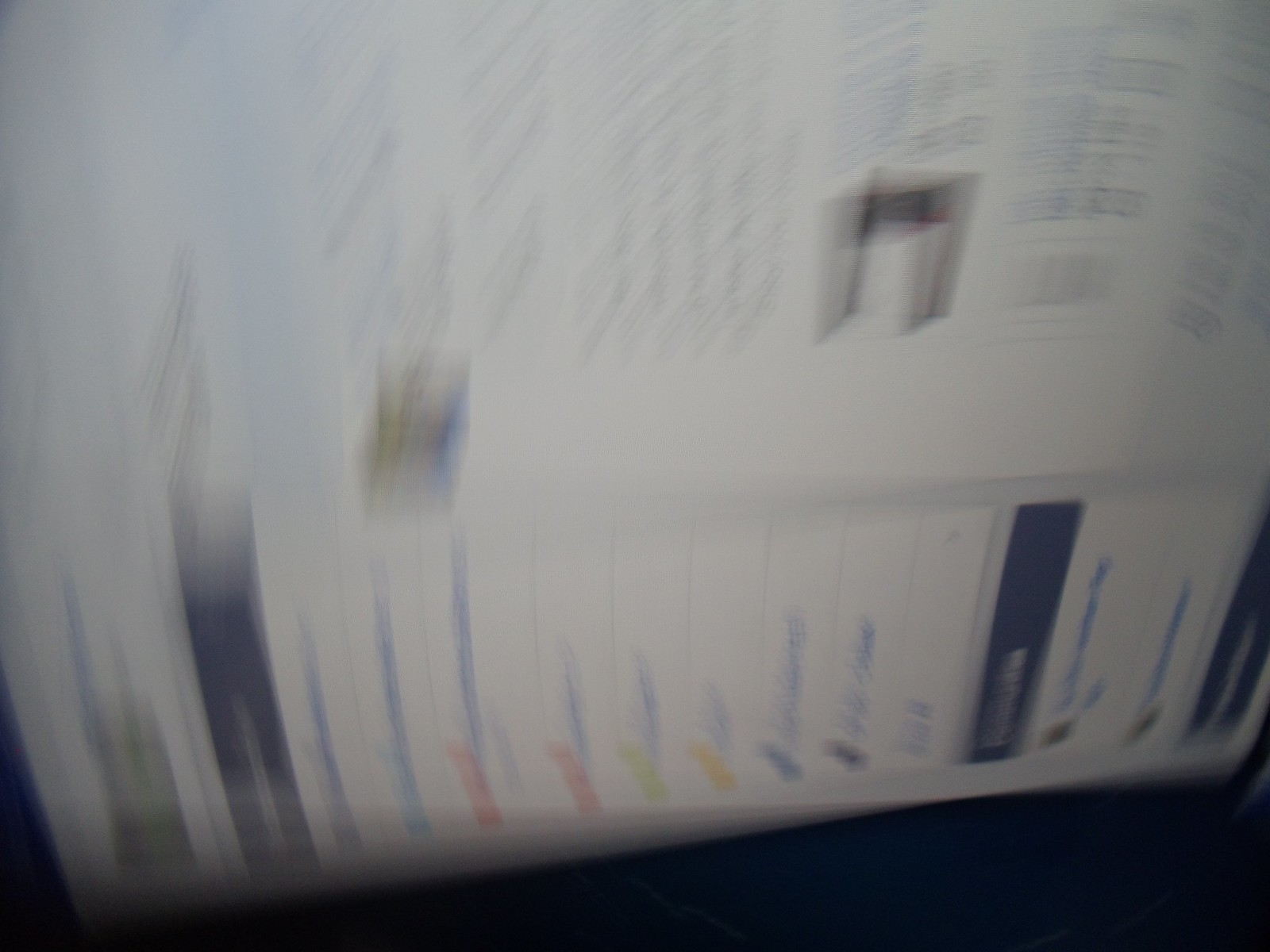The image depicts a blurry photograph of a computer screen displaying an e-commerce website. The photo seems to have been taken hastily and is oriented sideways. The interface includes a navigation panel on the left, which contains two sections. The first section features a list of names with icons adjacent to each entry, all under a navy blue header. The second, smaller section also has a navy header and includes two items. The main content area of the webpage showcases a typical e-commerce layout with two text boxes, blue hyperlinks, and a price list. The background color of the webpage is white.